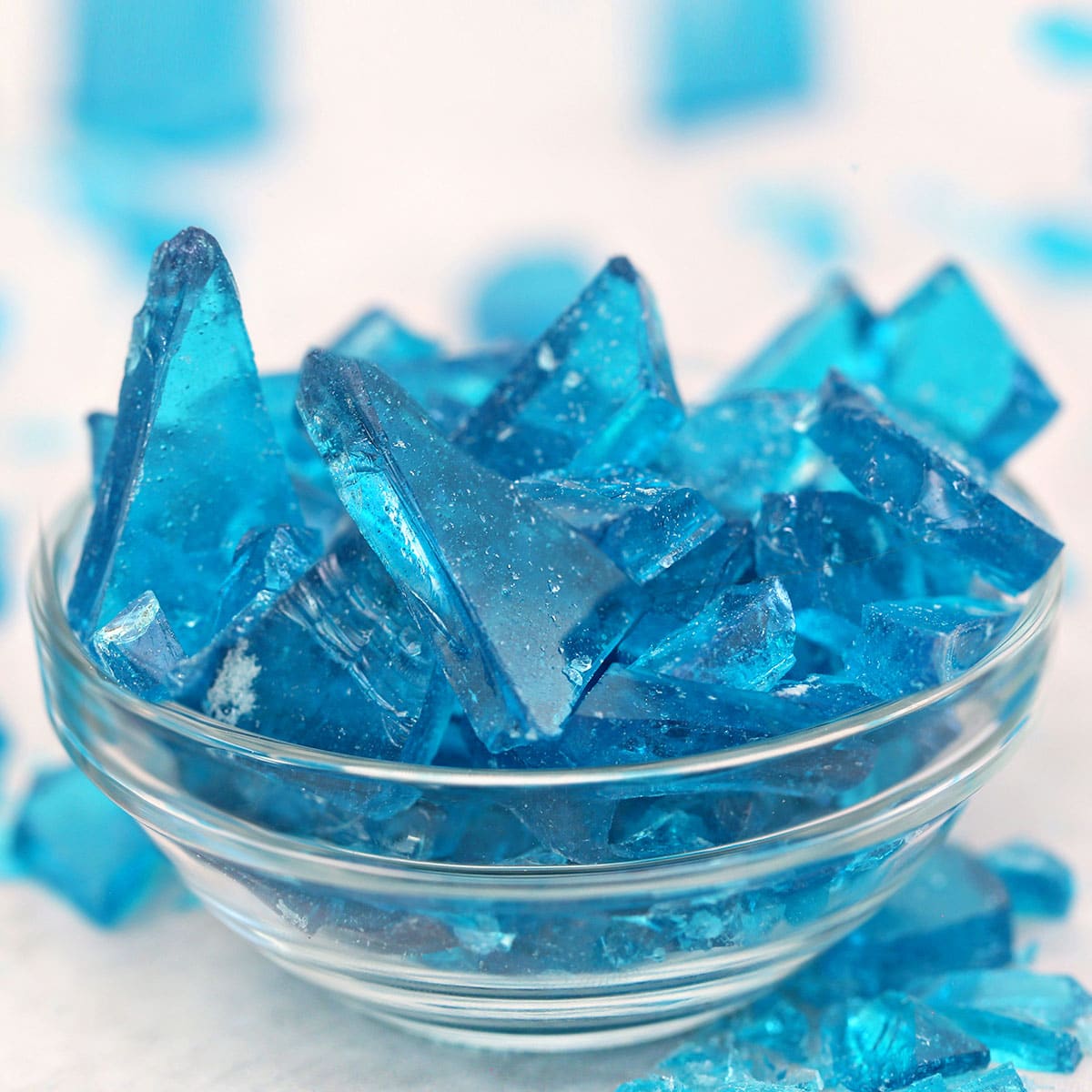The picture showcases a clear glass bowl with numerous ridges along its side, holding multiple striking blue crystals. These crystals, some with a triangular shape, scatter white flecks throughout their structure. Inside the bowl are also small shavings of these blue crystals, adding texture and depth. The background of the image is predominantly white, dotted with small, blurry, similarly colored crystals, emphasizing the vibrant blue hue and intricate nature of the contents. The overall effect makes the image intriguing and visually captivating, with its play on transparency, color, and light.